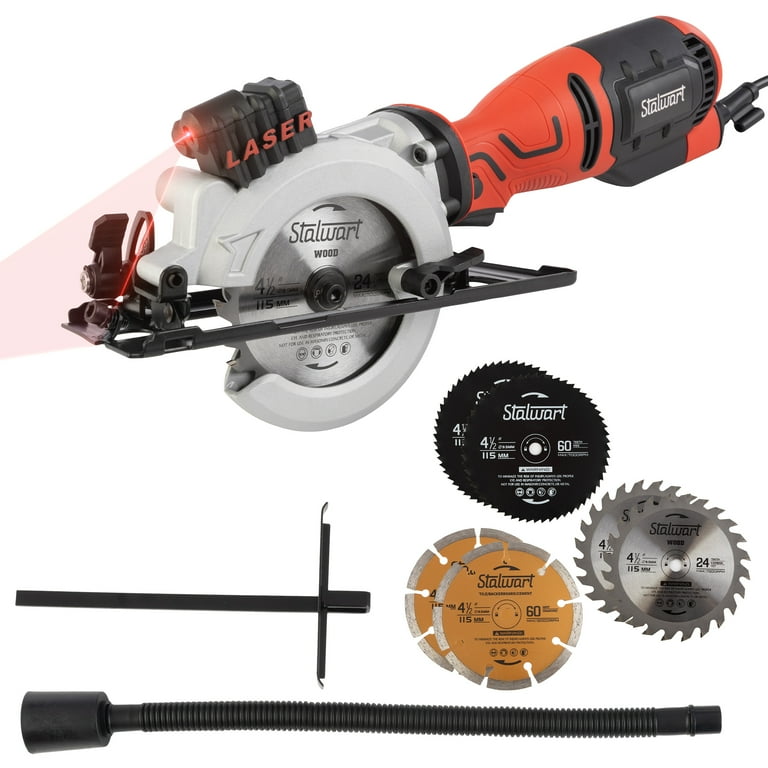This image features a compact, portable, corded electric circular saw by Stalwart, displayed against a pristine white background, likely intended for a product listing. The saw, designed for precise and versatile cutting tasks, especially in tight spaces, has an orange handle with a black safety bar and clearly marked "Stalwart" branding on its body. Attached to the saw is a standard 4.5-inch circular blade, labeled "Stalwart Wood," with some smaller, unreadable text.

A distinctive feature of this saw is its integrated laser guide system, evidenced by a black laser attachment that emits a red laser beam, aiding in precise cutting alignments. This attachment is prominently marked with the word "Laser."

Included in the lower part of the image are a series of six additional circular saw blades in varying styles: two black, two silver, and two with a yellow and silver combination, all matching the 4.5-inch size specification. Accompanying these blades are supplementary accessories: a sturdy plastic tube, potentially for dust collection or storage, a metal device which could be interpreted as a hanger for convenient storage, a T-shaped wrench for blade installation, and a cord strain protector, emphasizing the product’s comprehensive utility and accessories.